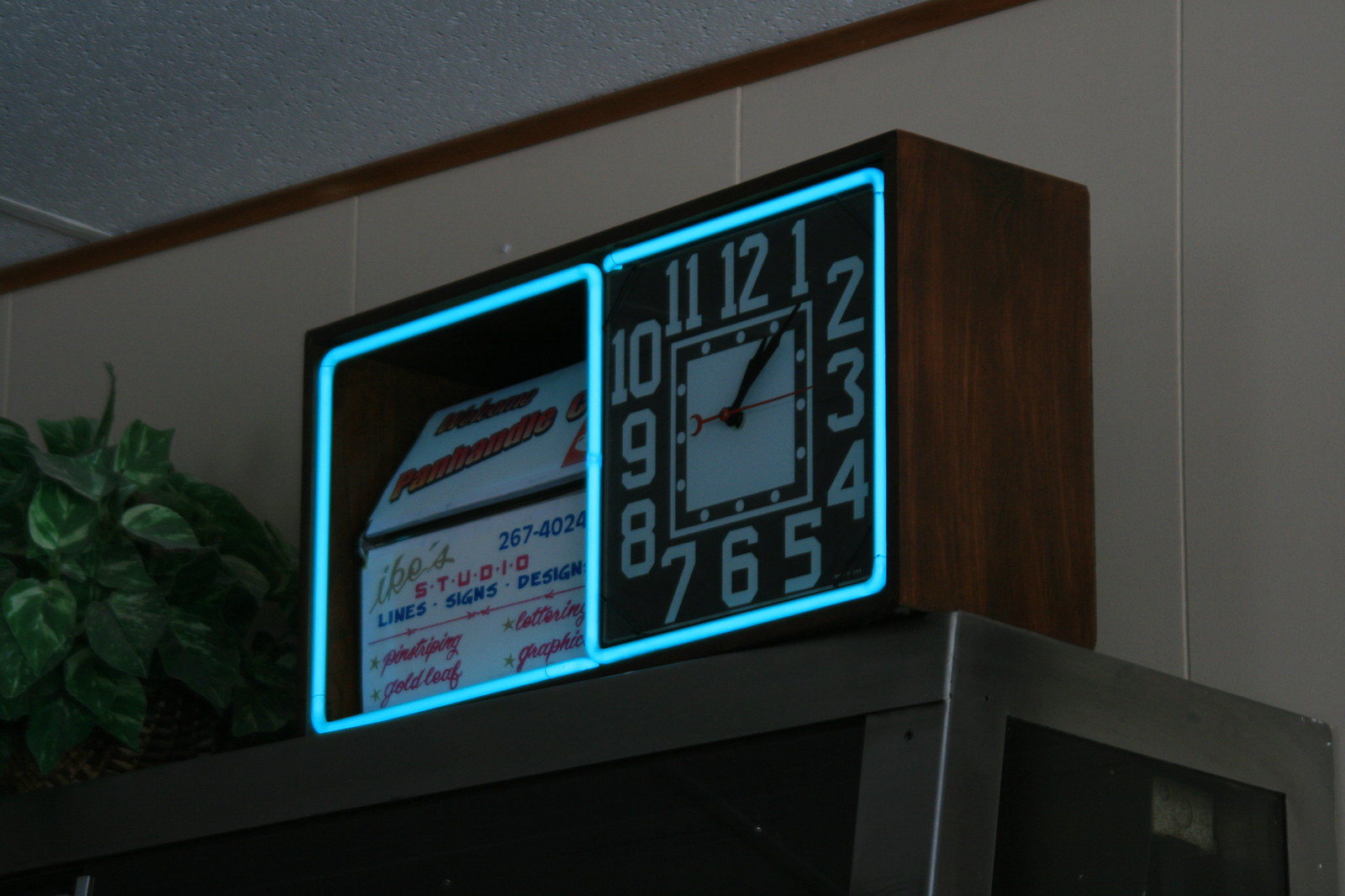In this image, a square-shaped clock is prominently displayed inside a rectangular brown shelving unit. The unit itself is situated on a high platform, the upper part of which is visible and is colored in shades of gray and black. The right and top sides of this structure are dark brown. The clock, positioned on the right side of the shelving unit, features a light blue square illumination around its face. The clock dial displays all the numbers from 1 to 12 in gray, with both black hands pointing to 1. On the left side of the shelving unit, a couple of signs with blue and red text are visible. The background showcases a gray wall and a single greenhouse plant to the left of the clock structure. The ceiling above is also gray, adding to the overall muted color palette of the scene.